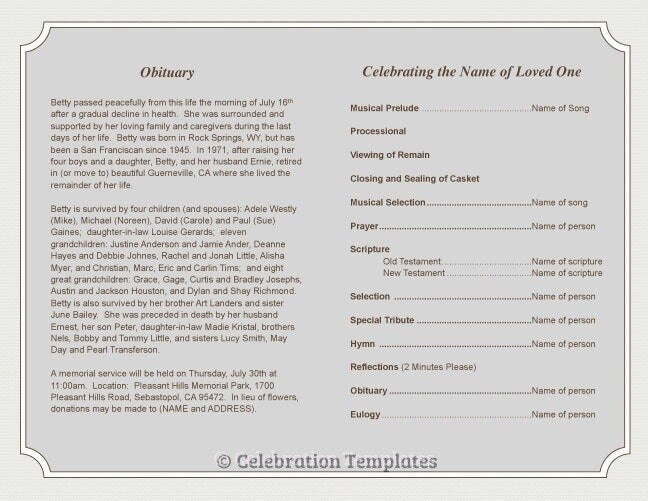The image depicts a black-and-white, landscape-oriented template for an obituary and ceremony. The document, set against a light gray background with clipped, curved corners, features a clean, structured layout with a white margin around the border. 

On the left side, the top-center header reads "Obituary" in bold black italics. Below this header are three paragraphs detailing the obituary of a woman named Betty. The first paragraph outlines the circumstances of her death and key aspects of her life, the middle paragraph lists her surviving relatives, and the final paragraph provides details about the upcoming memorial service.

The right side of the document is headed with "Celebrating the Name of Loved One" in bold black italics. It outlines various parts of the ceremonial process, including a musical prelude, a processional, viewing of remains, closing and sealing of the casket, additional musical selections, prayers, scripture readings from both the Old and New Testaments, a special tribute, a hymn, reflections, and a eulogy. 

The bottom of the document features a watermark reading "Celebration Templates." Despite its somber content, the template's design is elegant, with clear black text on a light gray background, suitable for a fitting tribute.